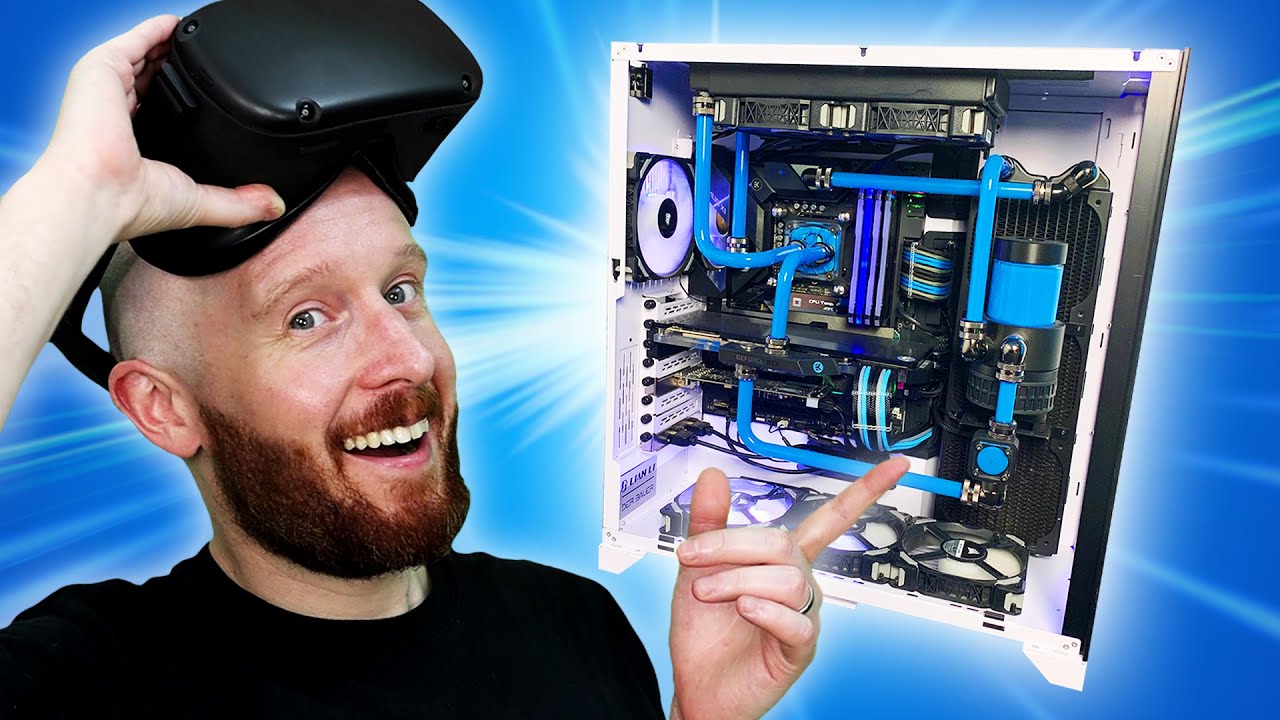This color photograph, likely a thumbnail for a YouTube video, features a bald, middle-aged white man with a short red beard and mustache. He is positioned on the left side of the image and is facing towards the right. He is wearing a black t-shirt and holding up a nondescript black VR headset over his forehead with his right hand. His left hand is extended, pointing at an open desktop gaming PC on the right side of the image. The PC, which has its side panel removed, reveals intricately arranged black components and bright blue cooling tubes. The background showcases a gradient blue backdrop with a white starburst pattern radiating from behind the computer. The man, smiling broadly with his mouth open and eyes directed at the camera, appears to be excitedly presenting the PC's interior, which also includes a CD drive and cooling fans.